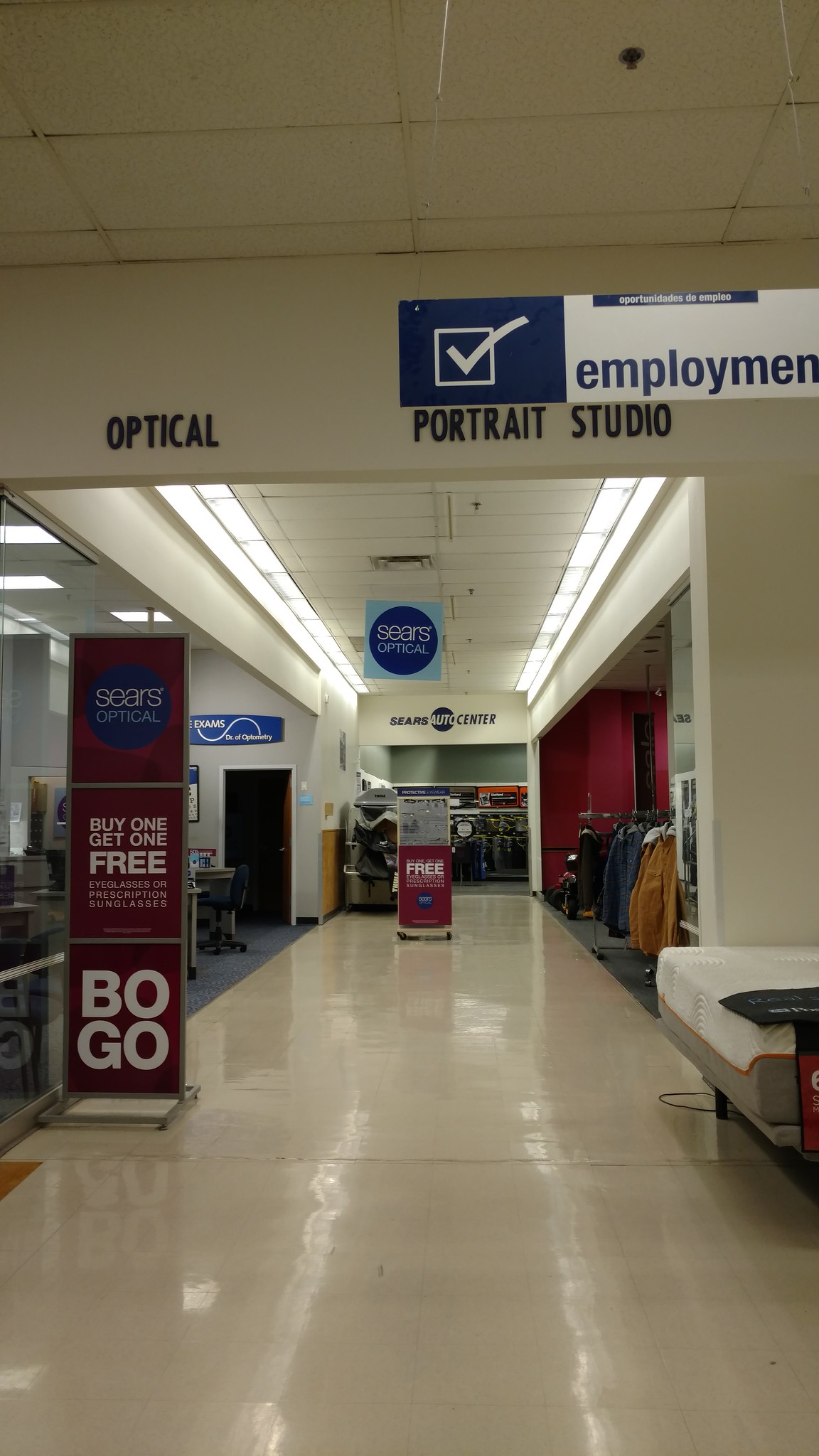This image depicts a commercial interior designed to resemble a hospital corridor. The setting features a long, wide corridor lined with a beige floor and illuminated by continuous strip lighting along the ceiling. On either side of the corridor, there are recessed niches, giving the space depth and function. One niche showcases a display of clothes, while another provides a seating area for visitors.

Dominating the visual field, a large sign with a bold red background commands attention with the acronym "B.O.G.O.," a recognizable retail term for "Buy One, Get One." Although the specifics of the offer are partially obscured, it is clear there is a promotional deal encouraging purchases. Another prominent red sign situated centrally in the corridor simply states "FREE," enhancing the sense of ongoing sales and promotions within this commercial space.

The overall vibe suggests both retail accessibility and a somewhat clinical aesthetic, blending to create a unique shopping environment focused on enticing deals.